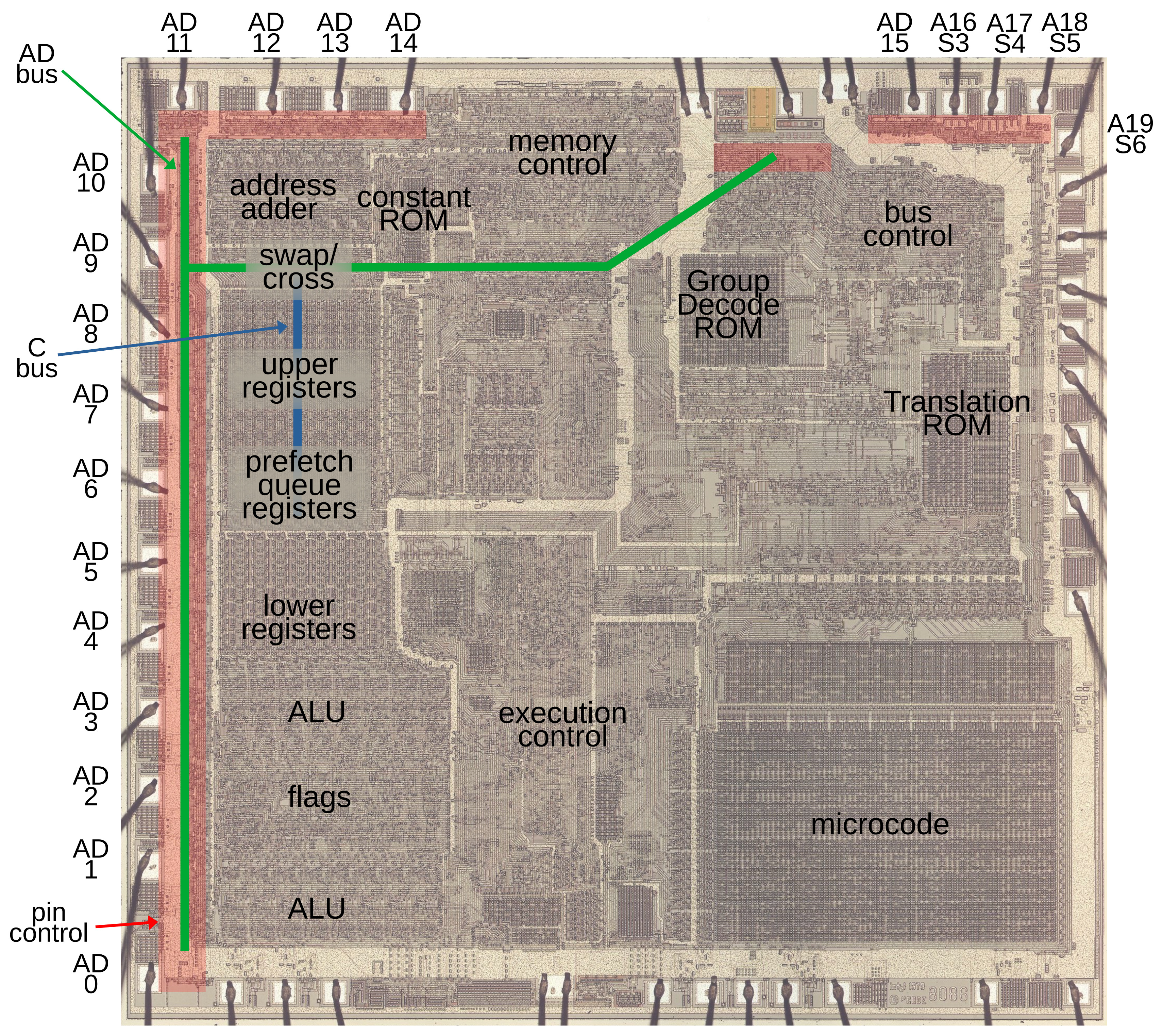This is a highly detailed diagram of an integrated circuit, resembling a vintage blueprint. The circuit is divided into blocks and squares, mostly in grey and yellow tones, with elements detailed in a purplish color. Each block is labeled with black text identifying components such as microcode, translation ROM, bus control, group decode ROM, memory control, constant ROM, address adder, swap cross, upper registers, prefetch queue registers, lower registers, ALU, and execution control. The border features numerous electrical diodes connected to rectangular white boxes labeled AD bus, AD10 through AD0 on one side, AD11 to AD14 on another, and AD15 to AD19, A16S3, A17S4, A18S5, A19S6 on the remaining sides. A green border line intersects the diagram, running through highlighted red areas which mark specific chip sections like the group decode ROM. The left side of the diagram emphasizes sections like the CBUS, swap cross, and prefetch queue registers, highlighted with a vertical blue bar and enclosed by a green borderline. The background of the diagram is white, enhancing the clarity and legibility of the details and labels.